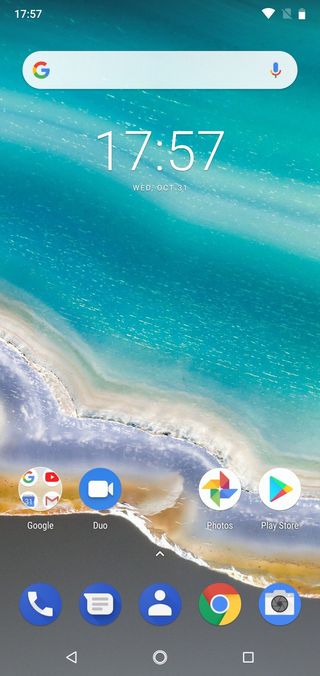The screenshot depicts a freshly started Android home screen, featuring a minimalist design with ample empty space. The wallpaper is an aerial view of a scenic coastline, showcasing a thin layer of sand leading into light blue water. As the view moves inland, the color transitions to a purplish-blue area, possibly depicting shallow water or wet sand, before turning into sand dunes and darker dirt.

At the top of the screen, a Google search bar is prominently placed, accompanied by a digital assistant icon. Below it, a clock widget displays the time, 17:57, in a 24-hour format alongside the date, Wednesday, October 31st.

The screen also features various app icons, with a folder grouping popular Google applications such as Assistant, YouTube, Calendar, and Gmail. Common apps like Duo, Photos, and the Play Store are present in the Dock, alongside essential tools such as Phone, Messages, Contacts, Chrome, and Camera. The overall layout is simple and uncluttered, allowing for ample customization and the addition of more apps or widgets.